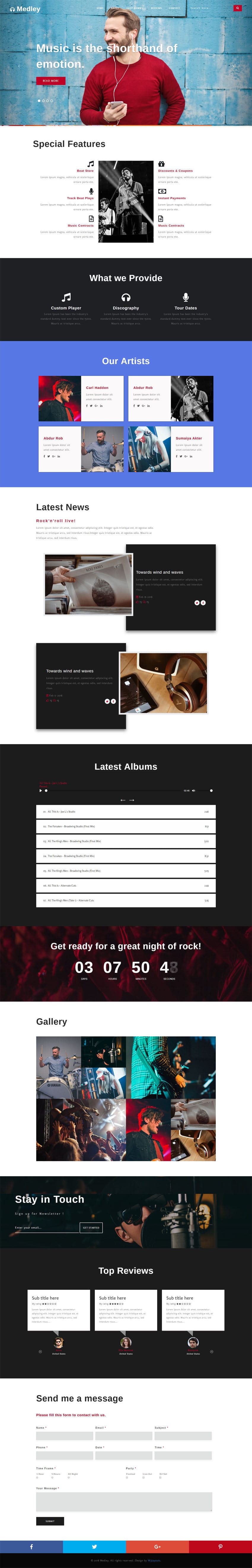The image displays a complex arrangement of nine stacked rectangular banners, each with varying background images and small text. 

At the topmost banner, there is an image of a bearded Caucasian man with short hair, wearing a long-sleeve red t-shirt. He appears to be against a partially faded blue-painted brick wall. The man is equipped with headphones and seems to be holding a phone. The text overlaying this image starts with "Music is the...", though the complete sentence is difficult to discern.

Below this is another banner featuring a predominantly black and white theme with shades of gray. It has the heading "Special Features." The specific details are unclear due to the small text size, but the background is white with black and light gray text.

The subsequent banner has a black bar at the top featuring three white icons or links. Below that are four boxed images with accompanying text, set against a bluish background.

Following this, there is a banner resembling a news website, potentially titled "Latest News." It contains four overlapping boxes, each featuring images and text. Two of these boxes have black backgrounds with white text, while the other two include images. The precise content of the images and text remains illegible.

Overall, the image is highly intricate, blending various banners and webpages with interspersed images and text that challenge readability.